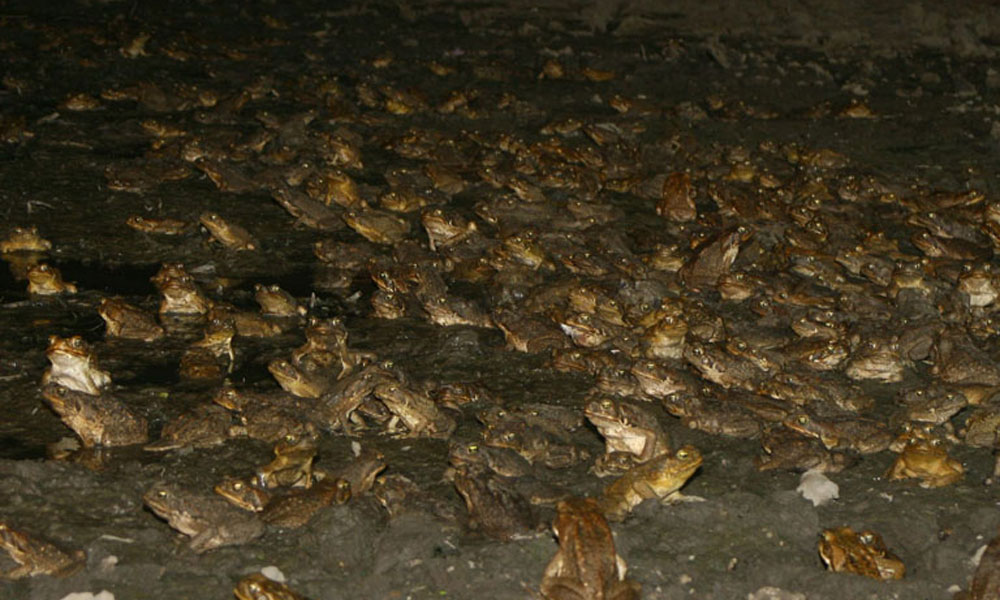This nighttime image captures a sprawling scene of what appears to be hundreds of frogs, densely populating a dark gray, muddy or rocky terrain. The frogs, in shades of dark brown, greenish-brown, and olive, exhibit lighter underbellies of off-white or pale yellow. Many frogs are clustered together, some seemingly mating, with individuals often layered on top of each other. The photograph, taken with a flash, highlights the frogs in the foreground with stark lighting, while those in the background fade into darkness. Their distinctive, shiny, and glowing eyes, positioned at various angles—some facing the camera, others looking sideways or away—create an almost surreal effect against the dim surroundings.